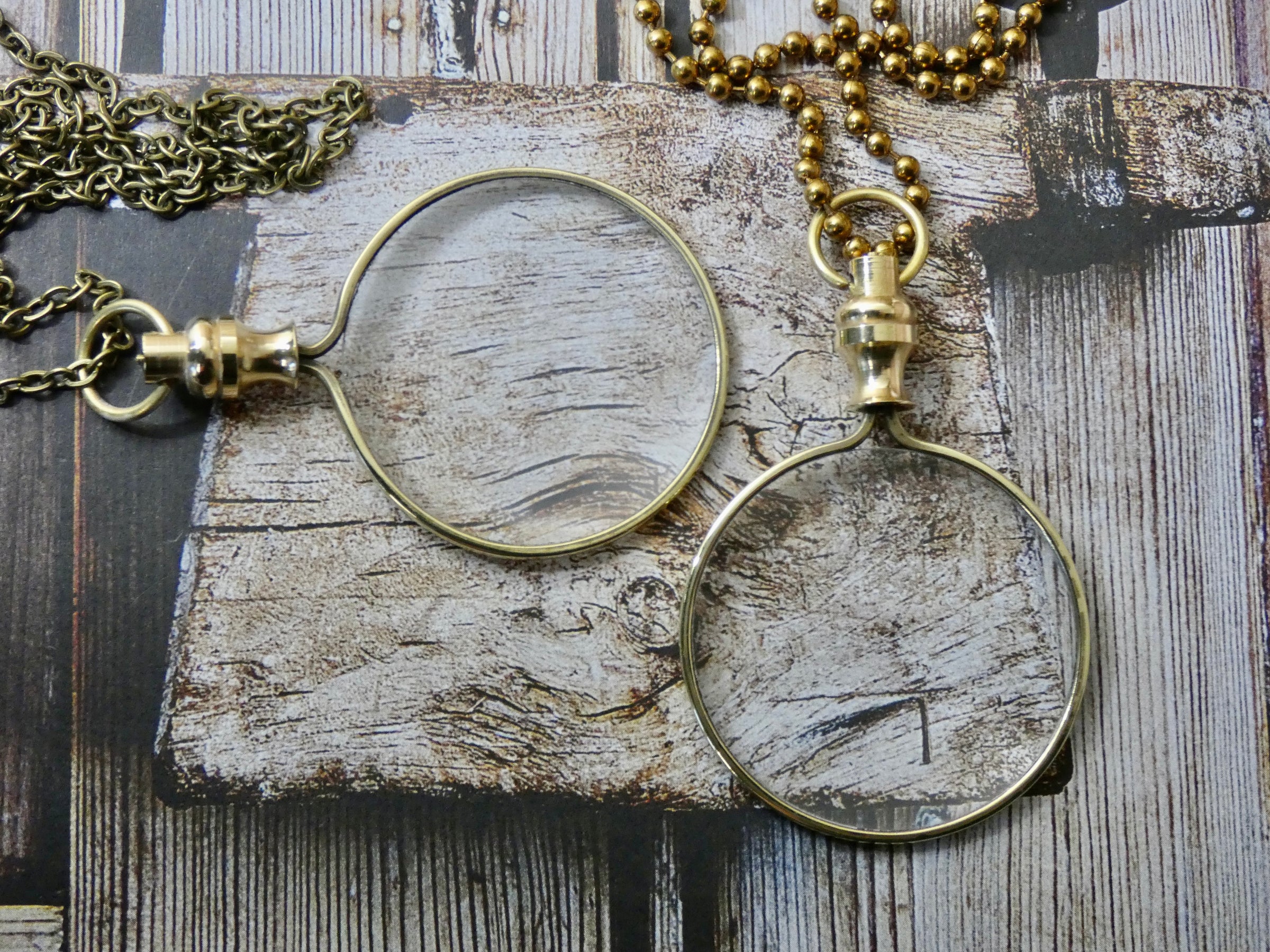The image captures two monocles with a vintage aesthetic, each featuring a circular design with a lens in the center. Both monocles are made from a copper-brass material, which matches the color of their chains. The monocle on the right is adorned with a beaded necklace chain, while the one on the left features a more traditional chain link necklace. These monocles are placed on a light grayish, distressed wooden surface that appears raw and untreated. The wood has distinct gaps and a rustic look, adding to the antique feel of the scene. The combination of these elements creates a cohesive and detailed display of vintage magnifying glasses.